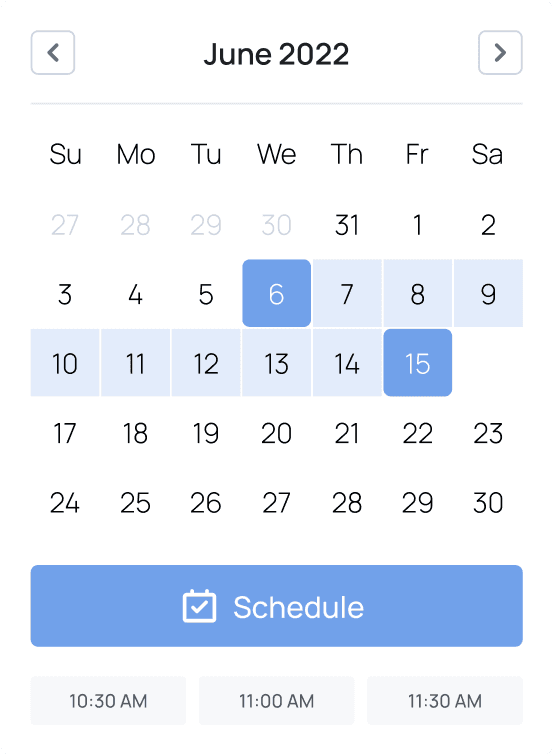The image is a screenshot taken from a tablet, possibly an iPad or a Samsung Galaxy Tablet. At the top of the screen, there's a navigational bar featuring an arrow and a square with rounded edges against a white background. At the center, the text "June 2022" is prominently displayed and perfectly centered. To the right, there is a smaller square icon containing an arrow pointing to the right.

Below this navigational bar, a new section starts, displaying the days of the week abbreviated in two letters: SU, MO, TU, WE, TH, FR, and SA. The calendar begins with Sunday (SU) on the 27th and progresses to the 31st under Thursday (TH). The first day of the new month, Friday the 1st, continues through to the 30th.

A series of dates from the 6th to the 15th are highlighted in blue. Specifically, the 6th and the 15th are marked with a dark blue color, while the dates from the 7th to the 14th are in light blue.

Towards the bottom of the screen, there's a rectangular "Schedule" button featuring an icon that indicates a schedule. Following this, there are buttons labeled 10:30, 11:00, and 11:30, likely intended to pull up available time slots or appointments. This detailed layout provides a comprehensive view of the highlighted dates and the interactive elements for scheduling.